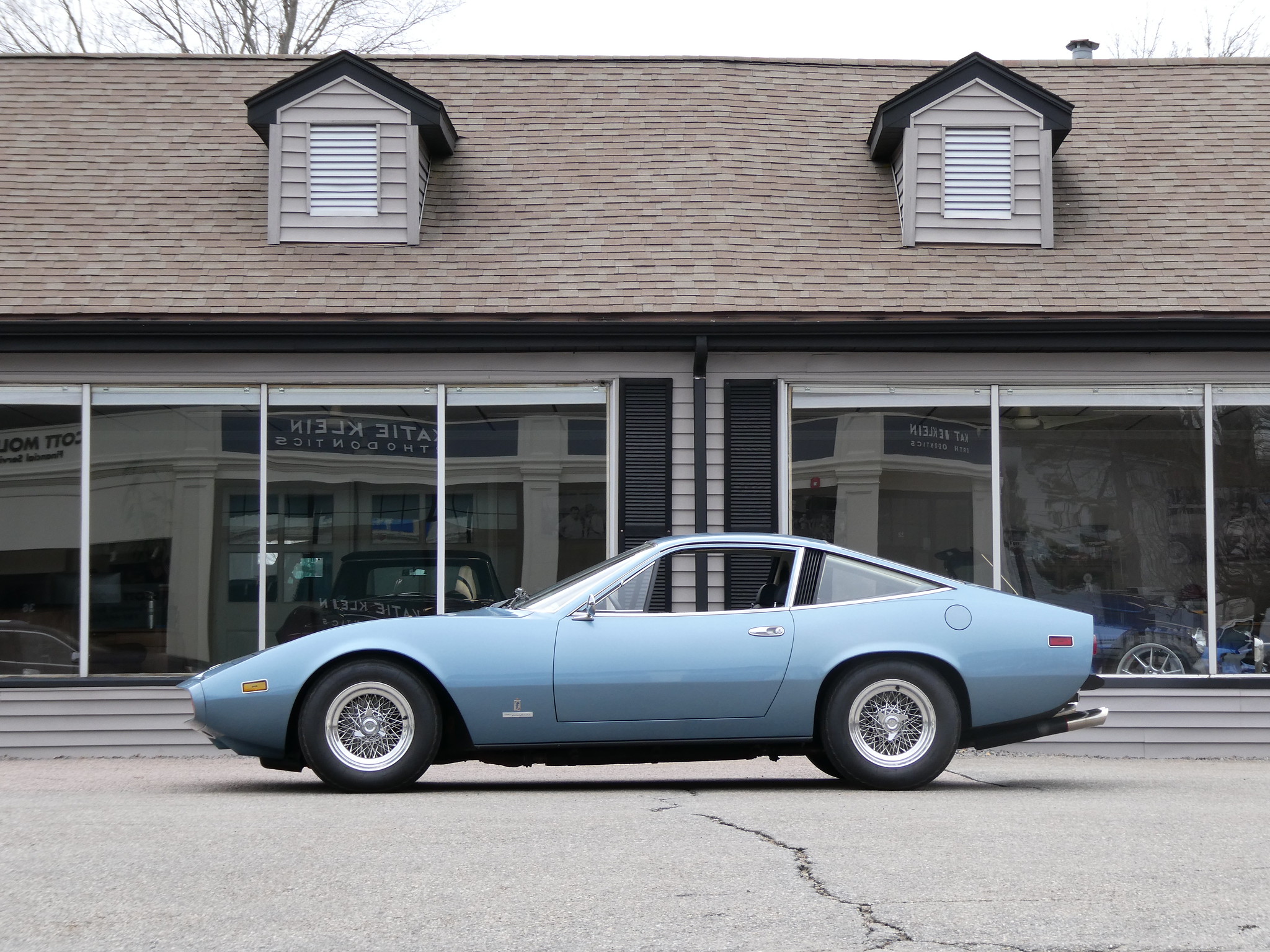The image captures a vintage light blue Corvette sports coupe, prominently positioned near the bottom center in a landscape orientation photograph. The car, recognized for its almost silver-blue hue, exudes classic charm with its sleek, aerodynamic design. Notable features include spoke tires with very thin spokes and metallic silver door handles. The vehicle has a distinct body shape with a sharply pointed back window, aligning in width with the front door window, complementing its sporty two-door structure.

In the reflections gleamed from its polished surface, a background story unfolds. The car is parked on a gray asphalt lot that resembles a parking area, complete with visible cracks enhancing its aged ambience. A single-story building with a low, light brown shingle roof and two prominent dormer windows forms the backdrop. The building's façade boasts clear glass windows running across its front, displaying older cars inside, adding to the nostalgic theme. White blinds are visible within the windows, and the structure is adorned with beige vinyl siding, black shutters, and a black gutter. The setting is further characterized by a white-gray sky and the bare silhouettes of trees, situating this vivid scene in a moment of quiet realism.